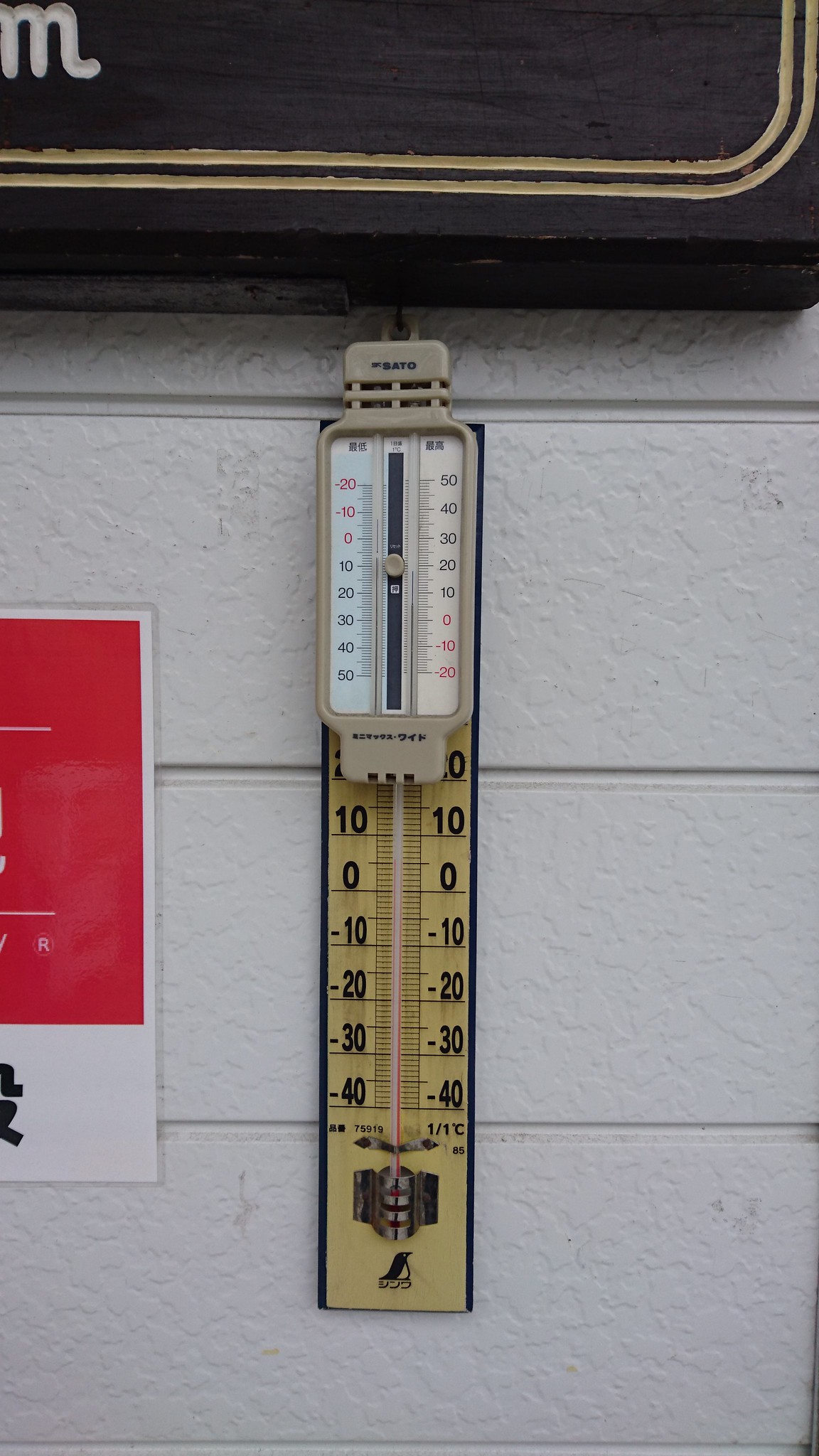This photograph captures a thermostat installed on a white stucco wall adorned with horizontal slats. The setting is ambiguous—it's challenging to discern whether it is indoor or outdoor. The stucco wall, divided into three distinct sections, serves as a backdrop for the centrally positioned thermostat. The device itself is composed of two parts: the upper half is white and features two distinct gauges, possibly indicating temperatures in Fahrenheit and Celsius. The gauges display black and red numbers, providing a clear readout.

Beneath this white thermostat is a yellowish component, reminiscent of the color of a classic wooden ruler. Adding a whimsical touch, a tiny penguin logo is visible at the bottom of the thermostat assembly. Enhancing the scene are two signs that frame the thermostat. Above it, only the bottom left corner of a wooden sign is visible. This sign is dark brown and features two thin, goldish stripes curving upward at its right edge, with the letter "M" in white inlaid into the wood.

To the left of the thermostat, a smaller sign is affixed—this one appearing as a white card with a red top section. Although the card bears black lettering, the text is not legible from this vantage point. The intricate details and surrounding elements make this seemingly mundane scene rich with texture and visual interest.